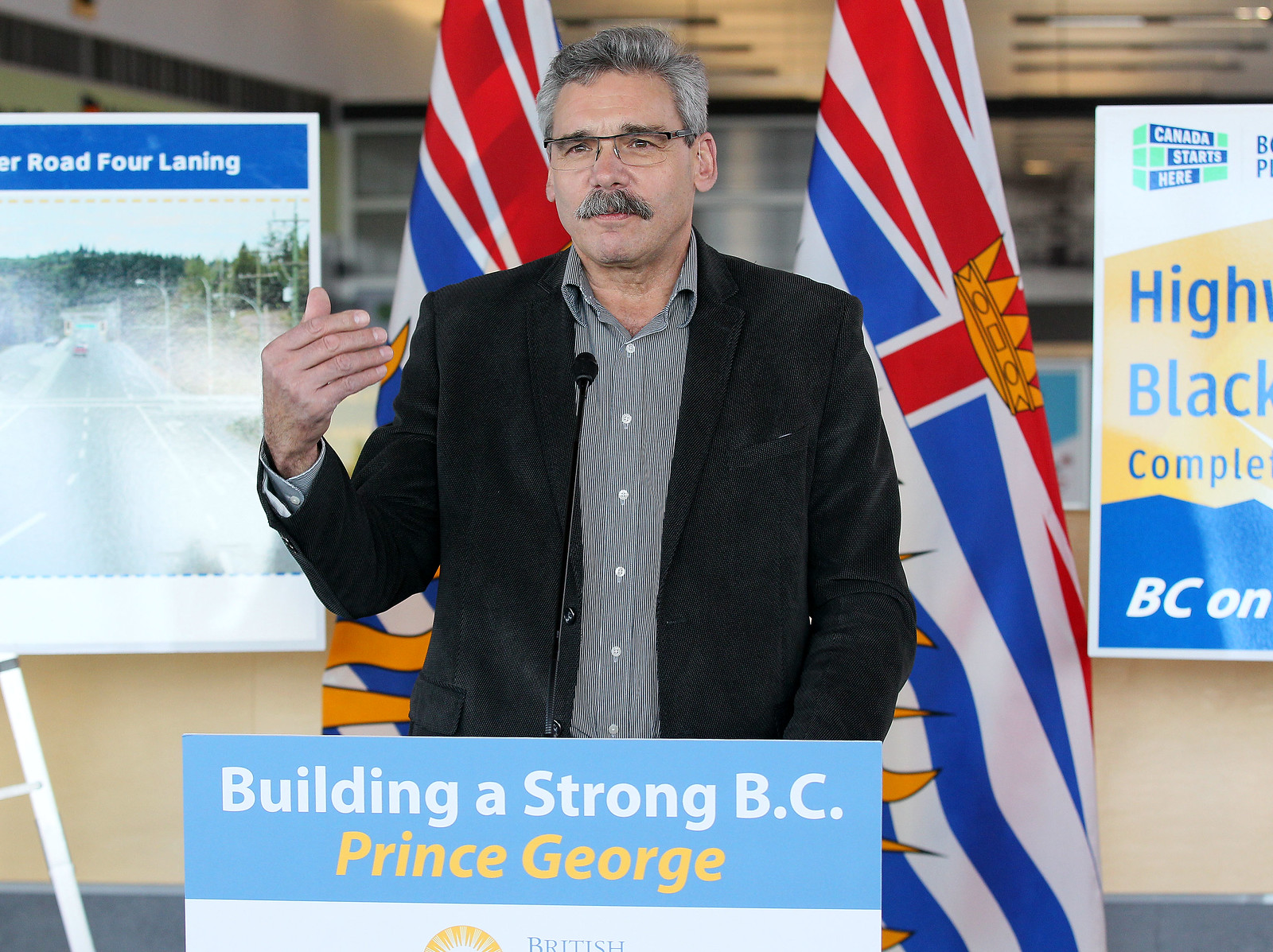The color photograph in landscape orientation features a distinguished man addressing an audience from a podium. The man, sporting salt and pepper hair, a mustache, and dark glasses, is clad in a black sport jacket over a gray-striped shirt. He is gesturing with his left hand while his right hand is raised, and he has a microphone on his lapel. The podium in front of him bears a sign that reads "Building a Strong BC" in white letters against a blue background, with "Prince George" written below in a yellow italic font.

Behind him, two flags with red, white, and blue stripes and hints of orange are prominently displayed, indicating a different nation's emblem. Flanking the podium on both sides are mounted posters related to his speech. On the right side, one poster shows a worn-out photograph with "Road 4 to Landing" on a blue background, and adjacent to it, another poster features a white background with "Hi Black" in yellow backing, and a blue portion with white lettering spelling "BC". The setting appears to be an interior hall, arranged for a formal gathering, possibly related to transportation or community development in Prince George, British Columbia, Canada.